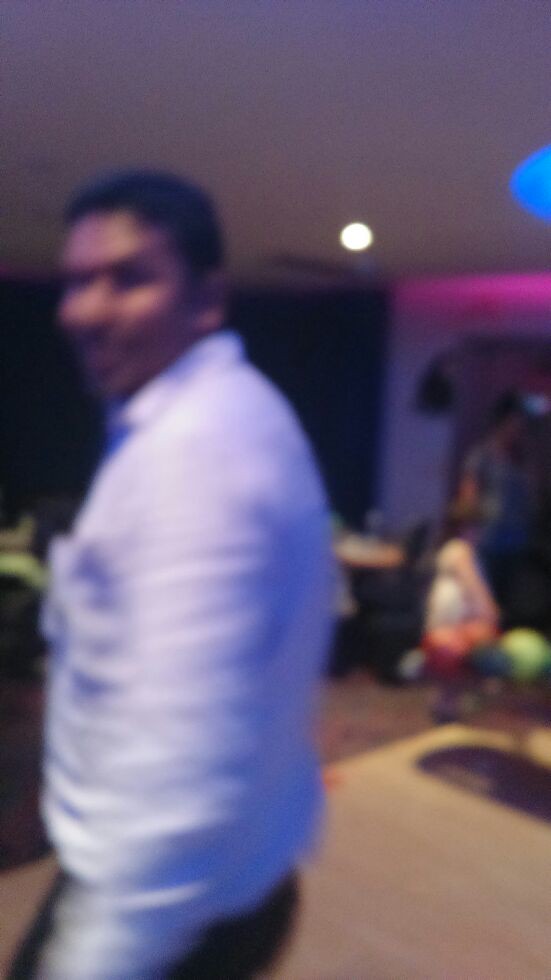The image depicts an adult male with dark skin and black hair, blurred to the extent that precise details are hard to discern. He is dressed in a light-colored shirt, possibly cream or white. His head is tilted towards the camera lens, although he appears to be moving to the left of the frame. The background features a room with a brown floor and a white ceiling, illuminated by overhead lighting. Scattered behind him are children’s toys, suggesting the setting might be a playroom or an area where children are present.